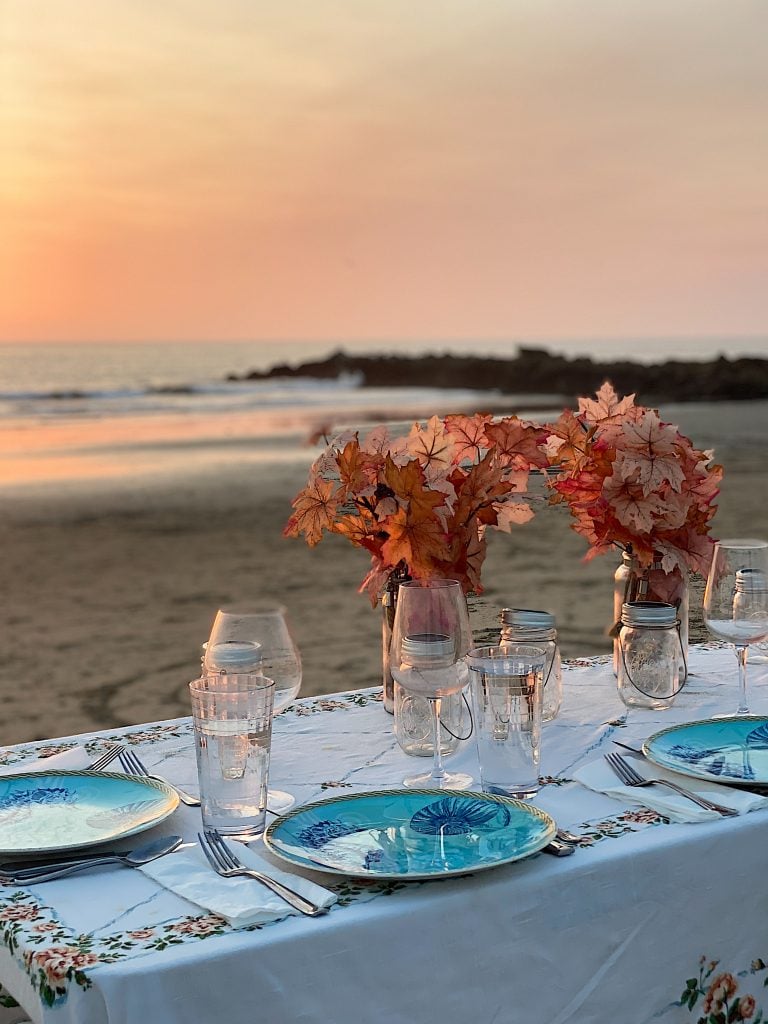Set against the scenic backdrop of a tranquil beach, the foreground is dominated by an elegantly set dining table, perfect for a sophisticated evening by the ocean. The setting sun casts an enchanting orange glow, illuminating the scene with a warm, romantic hue. The table is adorned with a pristine white tablecloth featuring an intricate floral print, adding a touch of delicate beauty to the arrangement.

The place settings are exquisite, featuring light blue china plates with elegant gold rims, each plate showcasing a captivating seashell design. The table is further embellished with polished silver cutlery and sparkling crystal wine glasses, complemented by intricately cut water glasses that catch the fading sunlight.

At the center of the table, mason jar vases filled with an artful assortment of dried red, brown, and cream-colored leaves serve as rustic yet sophisticated centerpieces. These autumnal hues add depth and texture to the setting, harmonizing perfectly with the beach's natural beauty.

In the sandy area surrounding the table, tire tracks are visible, hinting at recent activity by either a car or motorcycle, subtly reminding viewers of the dynamic interaction between nature and human presence in this idyllic coastal setting.